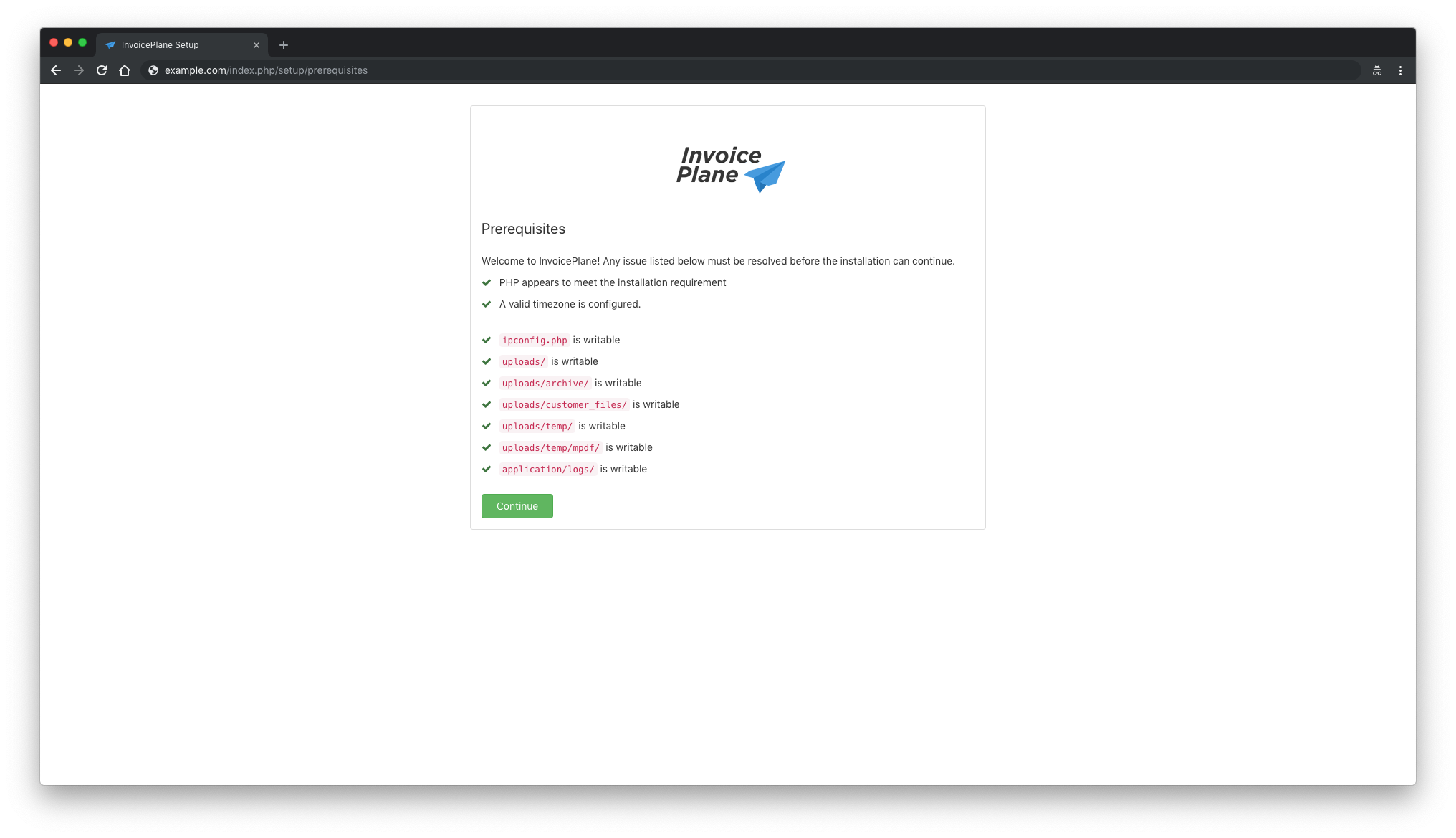The image depicts a computer monitor displaying a webpage in landscape orientation, with a notable length compared to its height. A prominent black bar spans across the top of the screen. In the top left corner of this bar, there are three small, horizontal buttons in red, yellow, and green, resembling a rotated traffic light. To the right of these buttons is some white text, presumably the website name, though it is not readable from the image. The black bar also contains several icons further to the right, ending with what appears to be a menu icon, accompanied by another indiscernible icon.

The main body of the screen is largely empty, with a plain white background. Centrally positioned is a fine gray line outlining a square containing the text "Invoice Plane" in black, italicized, Arial sans-serif font. Below this title is a blue, folded paper airplane logo representing the brand. Beneath the logo, the header "Prerequisites" is displayed, separated from subsequent text by a horizontal line.

Following this header, the text begins with a welcome message that is too small to read clearly. Below the welcome text, there are nine bulleted items, each marked with a green checkmark. The text of these items is in very tiny black font, with some portions appearing in red with pink highlighting, suggesting they are clickable links—seven such links are noticeable. At the bottom of this section, a green rectangular button is displayed, likely labeled with an action prompt such as "Get Started" or "Submit."